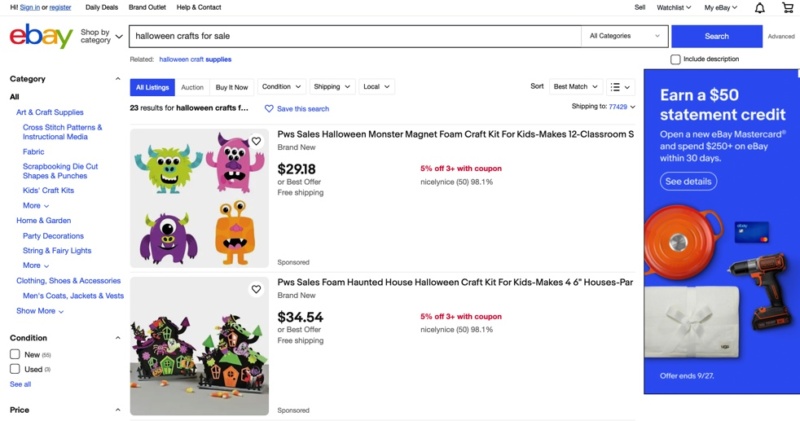This rectangular image is a screenshot of an eBay webpage. In the upper left corner, the eBay logo is displayed in its standard colors: red, blue, yellow, and green. Above the logo, there are small text links for "Hi, Sign in or register," "Daily Deals," "Brand Outlet," and "Help & Contact." On the right side of the header, the options "Sell," "Watch List," "My eBay," and a shopping cart icon are visible.

The main focus of the screenshot is on two listings in the "Arts and Craft Supplies" category. The first listing is for a "PWS Sales Halloween Monster Magnet Foam Craft Kit for Kids," which includes materials to make 12 classroom-sized crafts. The condition is brand-new, with a price of $29.18 or best offer, and free shipping. Additionally, there is a 5% discount available for purchases of three or more kits with a coupon. The seller, "Nicely Nice," has a feedback rating of 98.1%.

Beneath this listing is another similar one displaying two haunted house foam crafts. This is a "PWS Sales Foam Haunted House Halloween Craft Kit for Kids," priced at $34.54.